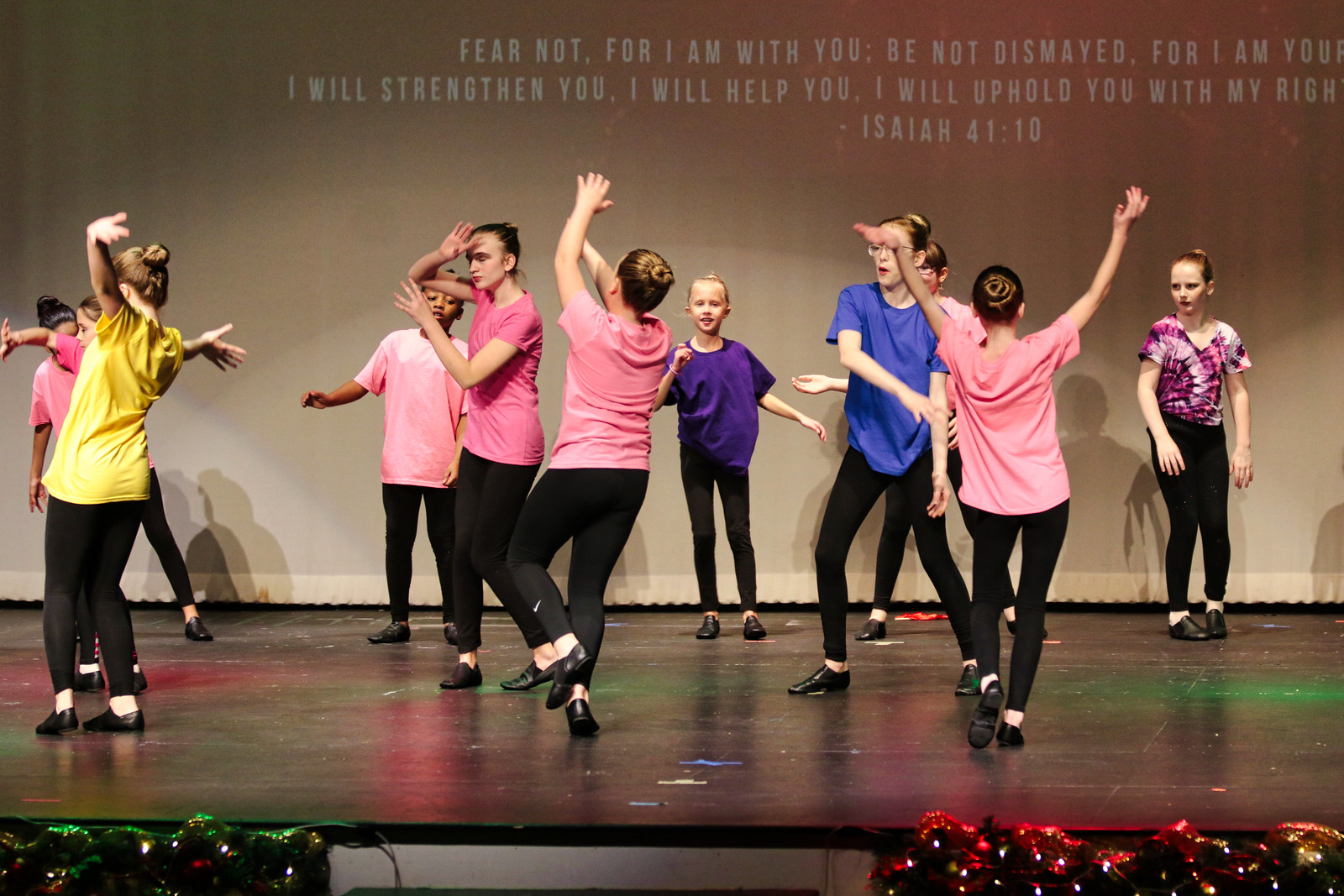In this vibrant photograph, a group of young female dancers, aged between 10 and 16, perform energetically on a black stage under multicolored lights. The girls, around a dozen in number, are dressed in an array of spring-colored t-shirts—pinks, purples, blues, and yellows—each paired with black leggings and flat, black leather dance shoes. Their dance movements are varied and spontaneous, with some girls reaching their arms upward while others stretch sideways. Behind them, a partially visible Biblical verse from Isaiah 41:10, written in white letters, reads: "Fear not, for I am with you. Be not dismayed, for I am... I will strengthen you. I will help you. I will uphold you with my right...". The dancers, consisting predominantly of Caucasian girls with two African Americans, exude joy and liveliness as they engage in what appears to be a joyous dance recital, each interpreting the rhythm in their unique way.